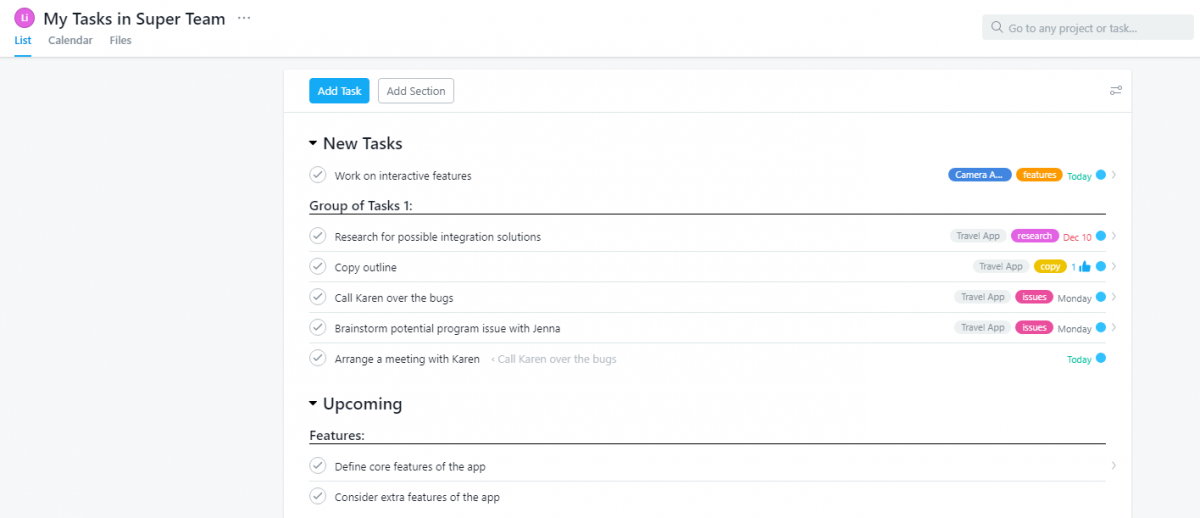**Detailed Caption:**

The screenshot depicts a task management page from a website interface. At the top left corner of the page, there is a white header featuring a pink circle containing the initials "Li" where "L" is capitalized and "i" is lowercase. Adjacent to this circle, a large bold black text reads "My Tasks in Superteam". On the far right of this, there are three horizontally aligned medium gray dots. Directly below this header section, the navigation is divided into three tabs: 

1. The first tab has blue text with a blue underlined list icon next to it.
2. The second tab labeled "Calendar" in gray text.
3. The third tab labeled "Files" in gray text.

To the far right of these tabs, after a considerable amount of empty white space, there is a medium gray search bar with the placeholder text "Go to any project or task" in dark gray text. Left of this search bar, there is a medium gray magnifying glass icon. Separating the header from the body of the page is a light gray horizontal line.

The body of the page beneath the header is light gray. Positioned in the center but slightly offset to the right, there is a prominent white rectangle with a thin light gray border. At the top left corner of this rectangle, there is a bright blue button with white text that says "Add Task." Directly to the right of the "Add Task" button, there is a white button outlined in light gray with gray text that says "Add Section." Below these buttons, a thin light gray line runs across the rectangle.

Within the main white portion of the rectangle, starting at the top left, a black downward-pointing arrow icon is positioned next to bold black text that says "New Tasks." Below this title, a gray check mark icon encased in a white circle with a light gray outline is visible, followed by the task label "Work on Interactive Features." 

Further down, the page is sectioned into various categories, each with a black header followed by a black underline. Each section contains lists of tasks, indicated by similar gray check mark icons next to descriptive labels.